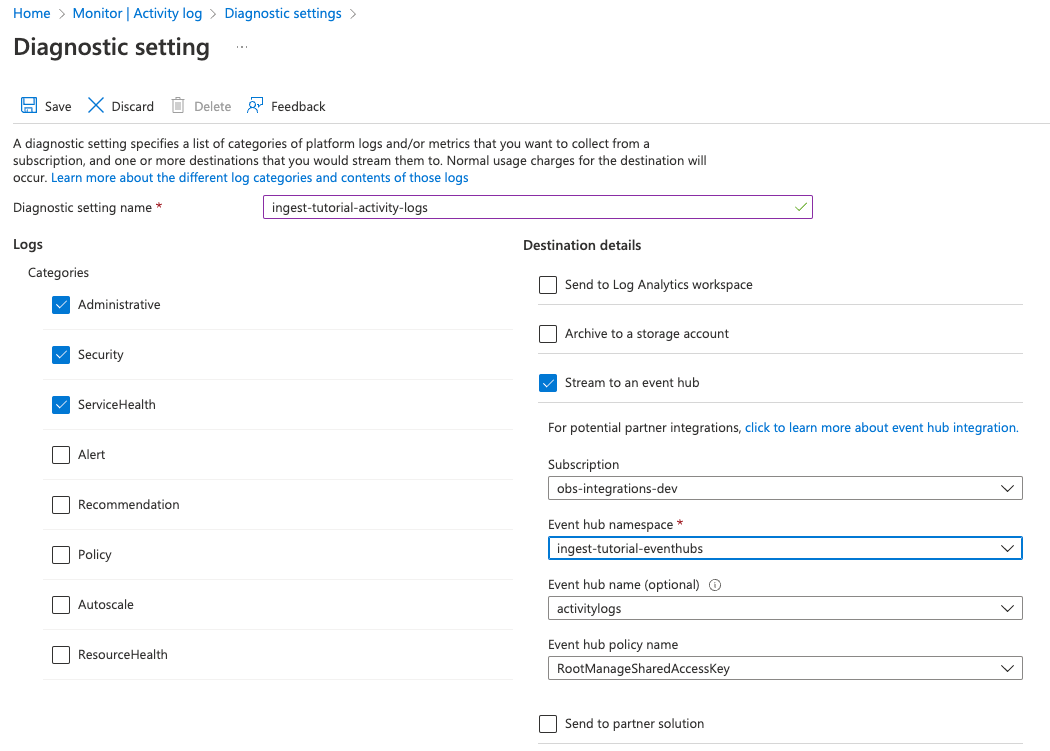The image is labeled "Diagnostic Setting" and serves as a detailed interface for configuring diagnostic settings. At the top of the page, there is a blue navigation bar that includes "Home," "Monitor Activity Log," and "Diagnostic Settings," each accompanied by arrows pointing to the right. Below this navigation bar, there are options for "Save," "Discard," "Delete," and "Feedback" related to the diagnostic settings.

A section describes that a diagnostic setting specifies a list of categories of platform logs and/or metrics to collect from a subscription, as well as one or more destinations to stream them to. It notes that normal usage charges for the destination will apply. There is also a link to learn more about the different log categories and their contents, highlighted in blue.

Under "Diagnostic Setting Name," marked with an asterisk indicating a required field, the name is "Ingest Tutorial Activity Logs." The logs are categorized into: Administrative, Security, Service, Health, Alert, Recommendation, Policy, Autoscale, and Resource Health.

On the right-hand side, the "Destination Details" section includes options to "Send to Log Analytics Workspace," "Archive to a Storage Account," and "Stream to an Event Hub." It mentions potential partner integrations and provides a clickable link to learn more about Event Hub integration.

Below this, there is a "Subscription" drop-down menu. "Event Hub Namespace," also marked with an asterisk, has its own drop-down menu. Additionally, there are fields for "Event Hub Name" (optional) and "Event Hub Policy Name." Lastly, there is an option to "Send to Partner Solution," which can be activated by checking a corresponding box.